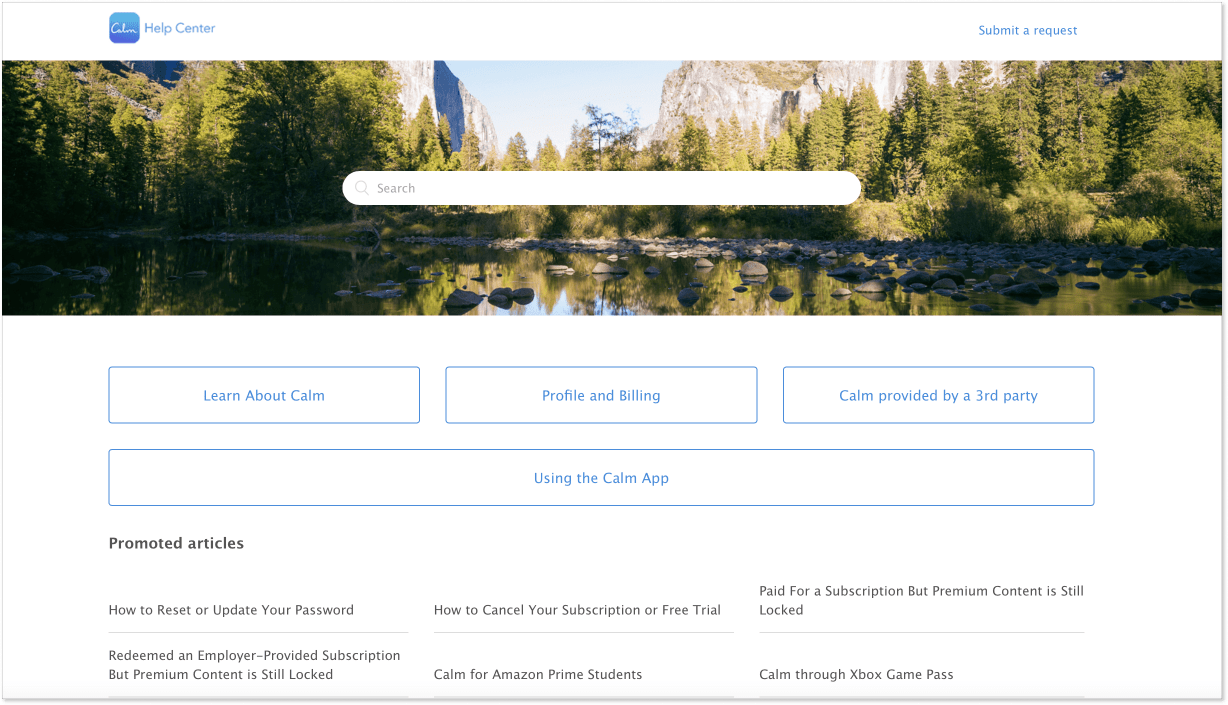The screenshot captures a web page from Calm's Help Center. The top section features a white banner. On the left side of the banner, there's a blue logo, likely square or rectangular, with the word "Calm" inside it. Next to the logo, in blue text, it reads "Help Center." On the right side of the banner, also in blue text, it says "Submit a Request."

Beneath the banner, a large panoramic image spans the entire width of the page, depicting a calm, serene lake surrounded by trees. Centered atop this image is a white search bar.

The background below the panoramic photo is white. This section is arranged with three rectangular boxes, each highlighted with blue outlines and containing blue text. From left to right, the boxes read: "Learn about Calm," "Profile and Billing," and "Calm Provided by a Third Party."

Below these three boxes is a large button that spans the same width, labeled "Using the Calm App."

Further down, in black text, a section titled "Promoted Articles" lists several help topics:
- How to reset or update your password
- Redeemed an employer-provided subscription but premium content is still locked
- How to cancel your subscription or free trial
- Calm for Amazon Prime students
- Paid for a subscription but premium content is still locked
- Calm through Xbox Game Pass.